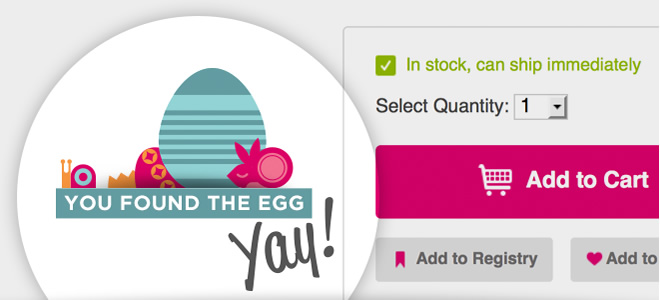In the image, the left side is dominated by a white circular area filled with various shapes and drawings. Toward the eastern section of this circle, there is a large, bluish egg adorned with blue stripes. To the right of the blue egg, a small cartoon rabbit, colored either red or pink, stands with a circular design inside its body. Adjacent to the giant blue egg is a small red egg, and on the far left, a snail is visible. Below these elements is a rectangular shape containing the text "You found the egg," with "Yay!" written in black at the bottom right corner.

On the right side of the image, set within a box, is a prominent rectangle displaying the phrase "Add to Cart" in white, accompanied by a shopping cart icon to its left. Below this rectangle, at the bottom right, are two buttons. The left button is labeled "Add to Registry" with a pink shopping tag icon to its left, while the right button is partially cut off, showing only "Add to" and a heart icon to its left. Above these buttons, the text "Select Quantity" is displayed with a counter set to "1." Further above, it states "In Stock - Can Ship Immediately."